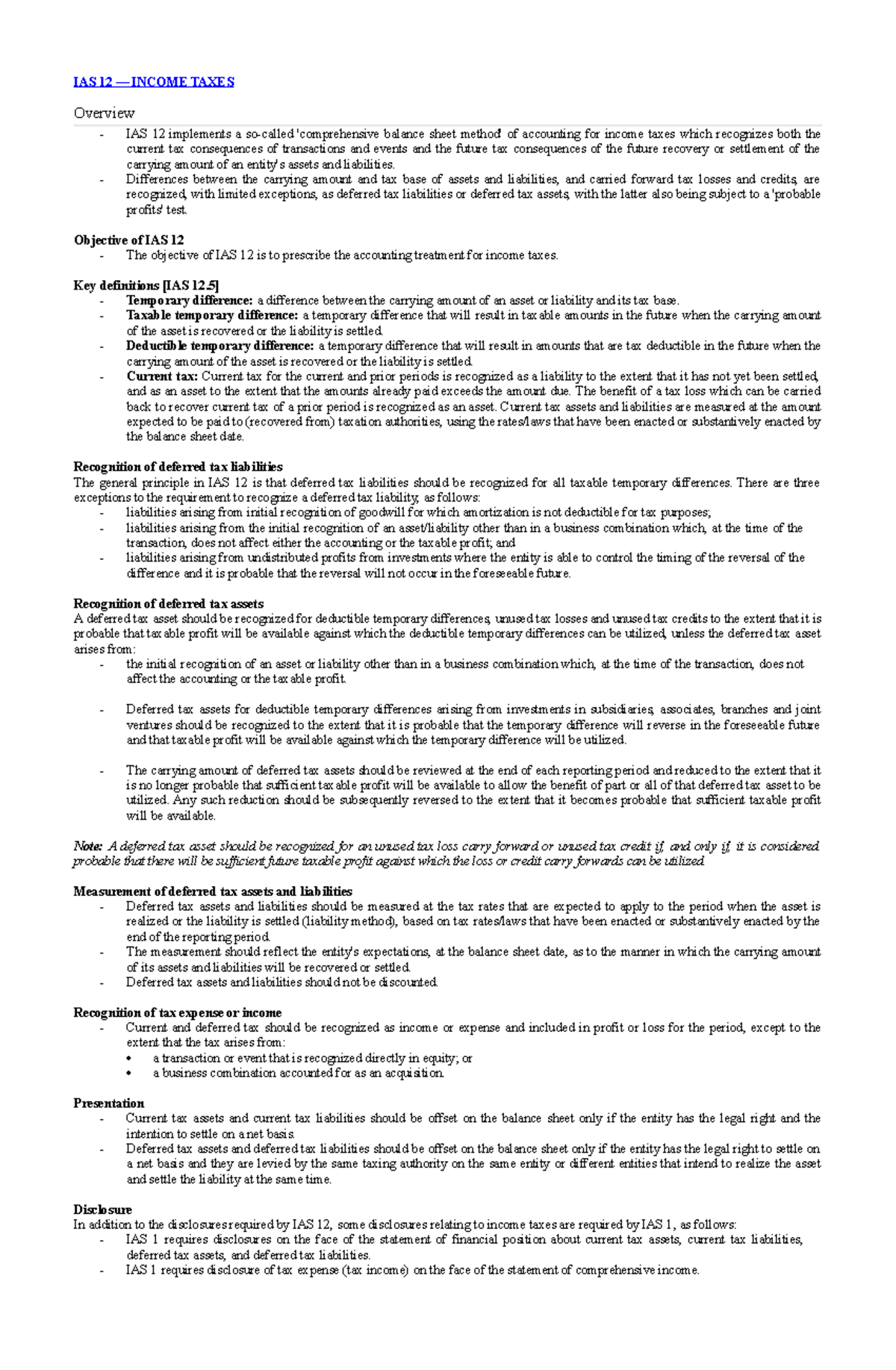The web page, predominantly styled in white with black text, features a clean and structured layout. At the top, the header "IAS 12 - Income Taxes" is prominently displayed in royal blue, underscored by a matching horizontal line. Following this header, the page is organized into a series of sections, each introduced by a subject heading.

The first section, "Overview," begins with two bullet points, providing a concise summary. Subsequent sections include "Objective of IAS 12," "Key Definitions," "Recognition of Deferred Tax Liabilities," "Recognition of Deferred Tax Assets," "Measurement of Deferred Tax Assets and Liabilities," "Recognition of Tax Expense or Income," "Presentation," and "Disclosure." 

Each section typically consists of a varying number of bullet points, and occasionally, a sentence or two of explanatory text precedes these lists. Furthermore, specific notes or additional clarifications are presented in italicized text to highlight important details or provide further context within each section. The layout ensures a comprehensive and easily navigable breakdown of IAS 12, facilitating the user's understanding of the topic.